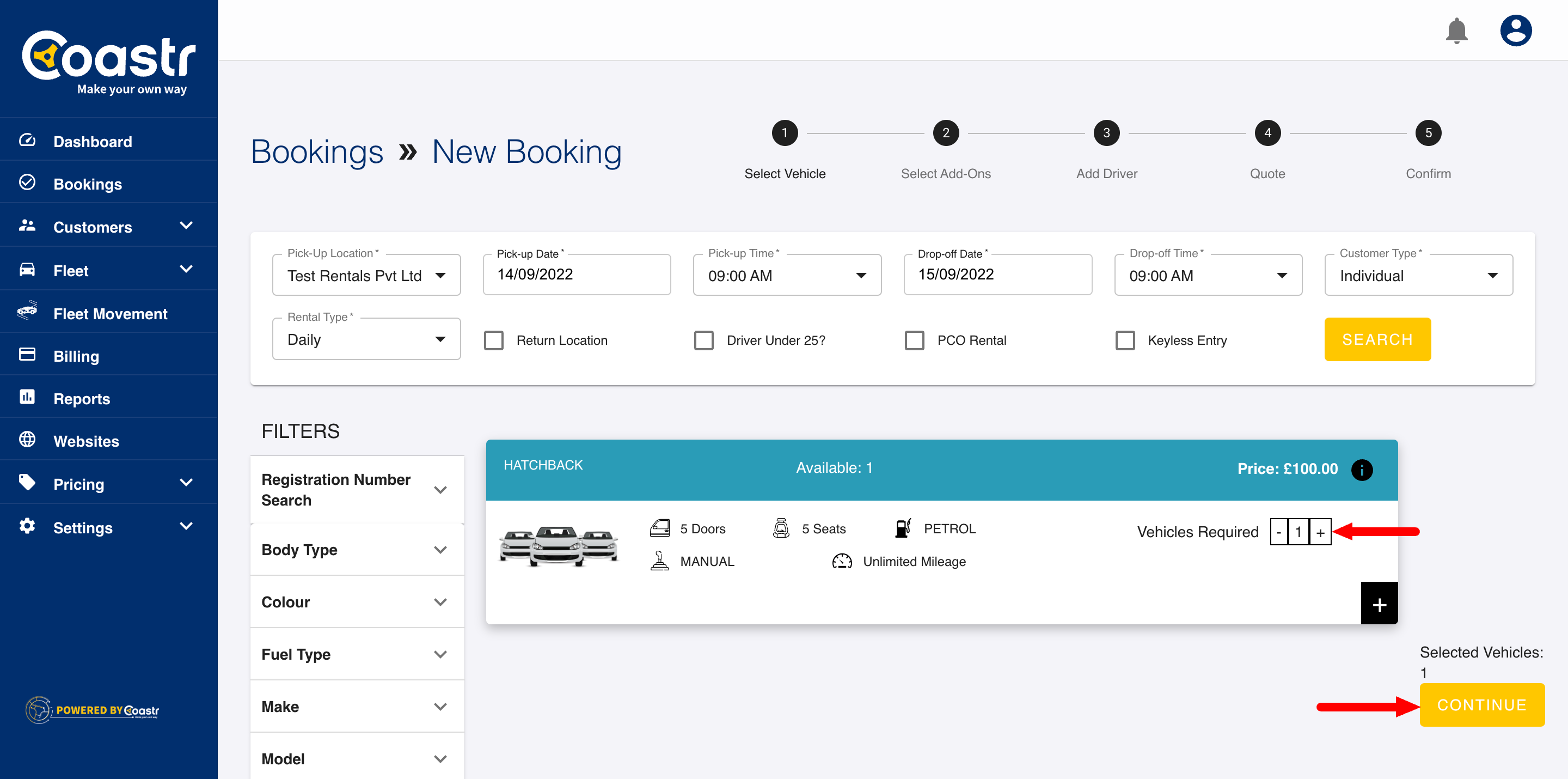This is a detailed cropped screenshot of the coaster booking page on the coaster website. 

### Left Panel:
- **Background Color:** Blue
- **Logo:** At the top in white
- **Tagline:** "Make your own way" in very small white letters, centered towards the right
- **Navigation Options:** 
  - Dashboard
  - Bookings
  - Customers
  - Fleet
  - Fleet Movement
  - Billing
  - Reports
  - Websites
  - Pricing
  - Settings
- **Footer:** Includes the coaster logo and "powered by Google"

### Main Section:
- **Background Color:** Gray
- **Header:** "Bookings, New Booking" in large blue letters at the top left
- **Options (Top Right of Header):**
  - Select Vehicle
  - Select Add-on
  - Add Driver
  - Add Quote
  - Custom
  - These options are connected by a very thin black line running from one to the next

### Booking Details Section:
- **Background Color:** White
- **Fields Listed:**
  - Booking details
  - Pickup location
  - Rental type
  - Pickup date
  - Pickup time
  - Drop-off date
  - Drop-off time
  - Customer type
  - Return location
  - Driver under 25
  - PCO rental
  - Keyless entry
- **Search Button:**
  - Color: Orange
  - Position: Right
  
### Filters Section:
- **Header:** "Filters" in large black letters
- **Fields Listed (Vertically):**
  - Registration number
  - Search
  - Body type
  - Color
  - Fuel type
  - Make
  - Model
  
### Vehicle Selection Section:
- **Header:** "Hatchback" in small white letters on a blue background
- **Available:** "1" in the center
- **Price:** "$100" to the right
- **Details:**
  - Bottom part of the box is white
  - Photo thumbnail: Front view of three white vehicles to the left
  - Features: Listed to the right of the thumbnail
  
### Vehicle Quantity Selection:
- **Label:** "Vehicles required"
- **Control:**
  - Number box showing "1"
  - Plus and minus buttons to adjust the quantity
- **Highlight:** A red arrow is edited onto the screenshot to highlight the "Vehicles required" section

### Continuation Button:
- **Color:** Orange
- **Label:** "Continue"
- **Highlight:** An arrow is edited onto the screenshot pointing directly at the "Continue" button at the bottom right